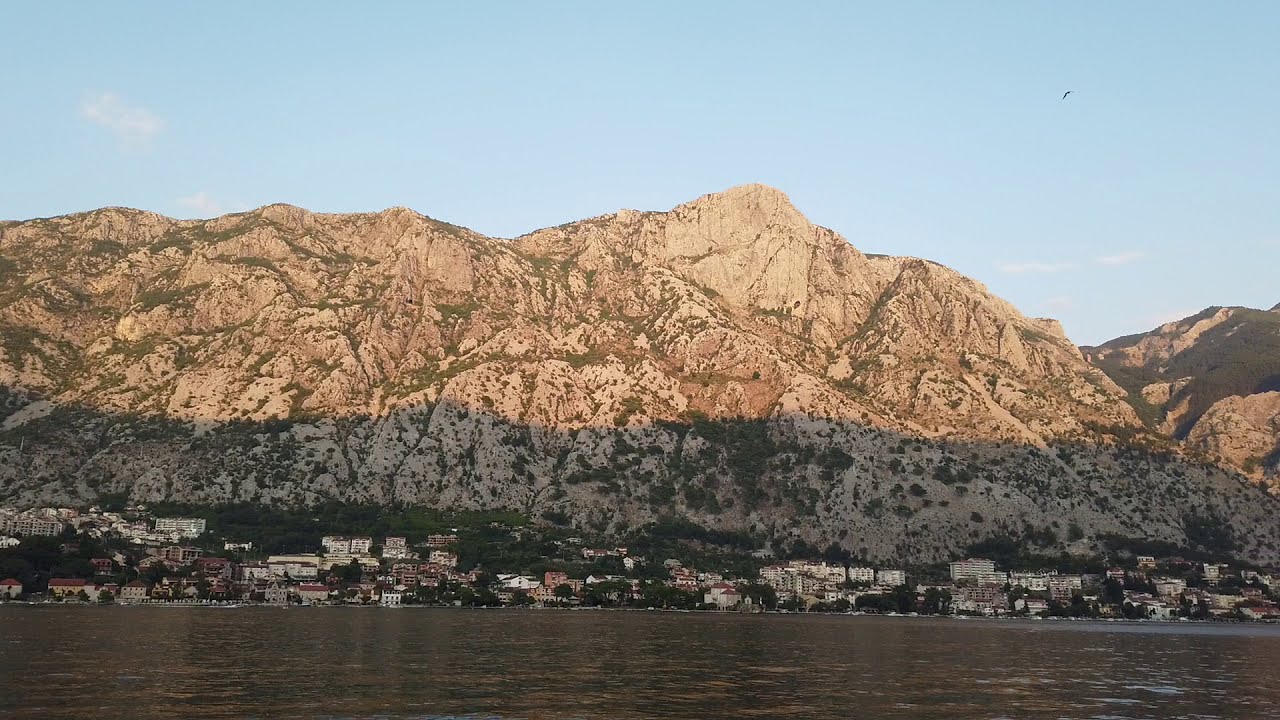The image captures a stunning large mountain landscape with a small town nestled at its foot, framed by a dark green and gray body of water in the foreground. The mountains, mostly tan and bare with sporadic green vegetation, rise high and cast shadows over half of their surface, suggesting a late time of day. Below the rugged peaks, numerous square and rectangular buildings with flat roofs lie scattered amidst various trees, giving the town a quaint, orderly appearance. These structures, primarily houses, are situated near the water's edge, some exhibiting tan or cream hues while others are brown. Docked boats are visible alongside these waterside dwellings, accentuating the town's connection to the water, which is relatively calm and brownish in color. The sky above is a clear light blue, dotted with a few small, white clouds, enhancing the serene and picturesque quality of the landscape.